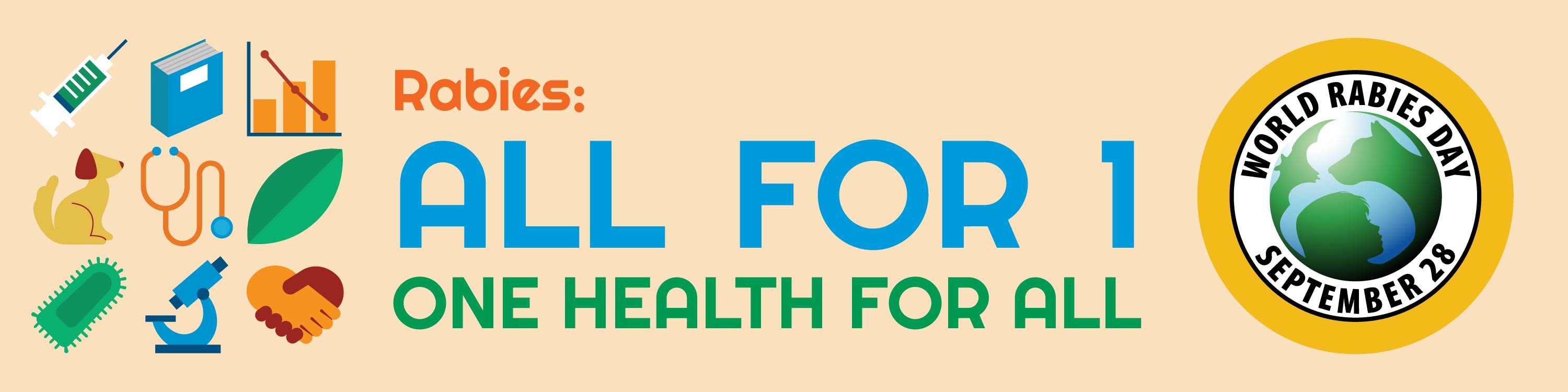The image is a digitally created promotional banner with a horizontally rectangular shape and no border, set against a pale pink or tan, bandaid-like background. On the far left are three rows of small clip art images, each with three icons: a hypodermic needle, a blue book, a bar graph, a sitting dog, a stethoscope, a green leaf, a green cell or bacteria, a blue microscope, and two shaking hands that form a heart. In the center of the banner, the text is arranged in three lines: the word "Rabies" in orange text with a colon, followed by "All for One" in large blue bold letters, and below it, "One Health for All" in green. On the right side, there is a seal featuring a yellow circle encircling a smaller white circle with a black rim that contains an image of a blue and green globe. Surrounding the globe, the text reads, "World Rabies Day" at the top and "September 28th" at the bottom. The banner incorporates various colors, including blue, green, yellow, orange, white, and tan.